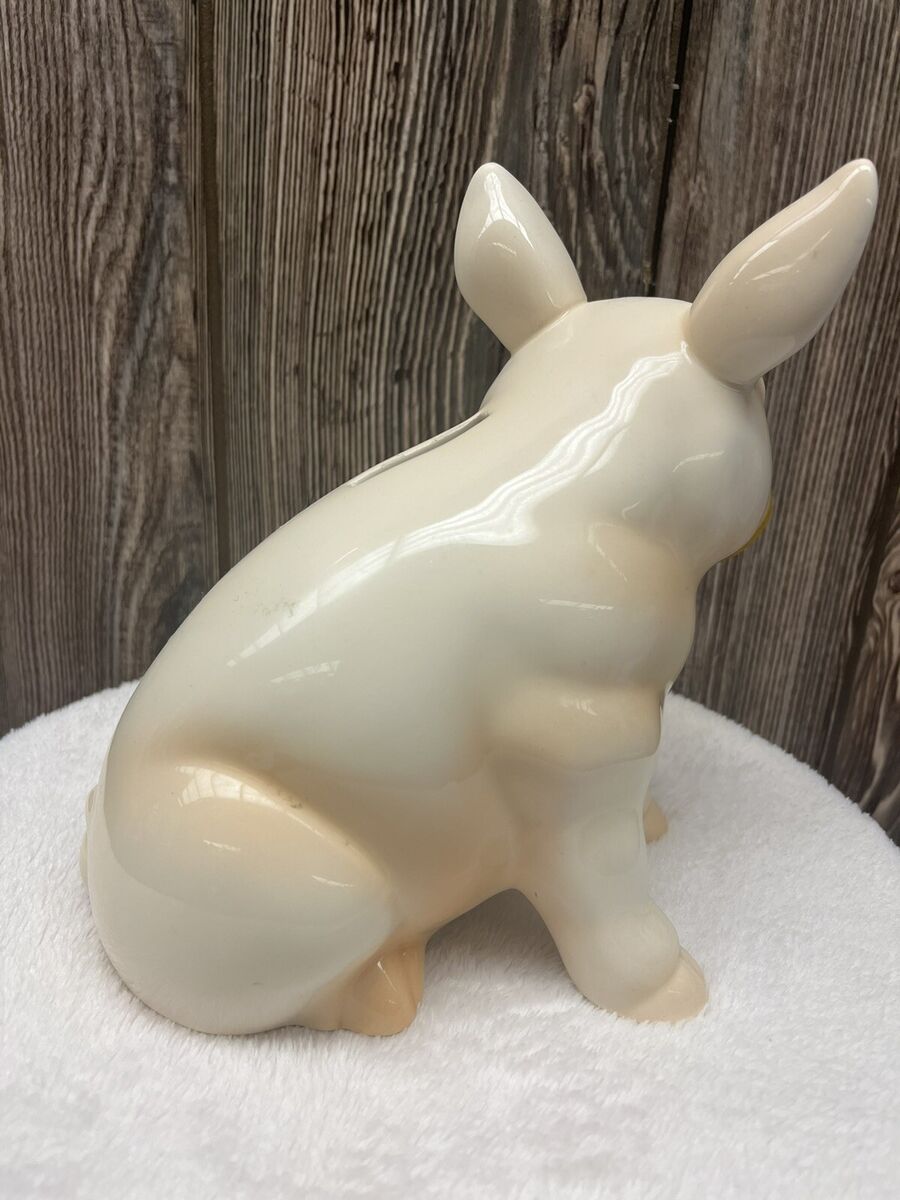In this vertically oriented photograph, a ceramic piggy bank, displaying a creamy whitish color with slight pinkish and brownish hues, is prominently featured. The piggy bank, characterized by its glossy finish, is facing away from the camera, revealing its distinct pig-like ears, front and back legs, and a coin slot on its back. It's seated on a white, fluffy, circular pad, resembling a fleece blanket, which is spread on a surface that could be a round table. Behind the piggy bank, a dark brown wooden wall composed of wooden planks forms the background, adding a rustic touch to the scene.